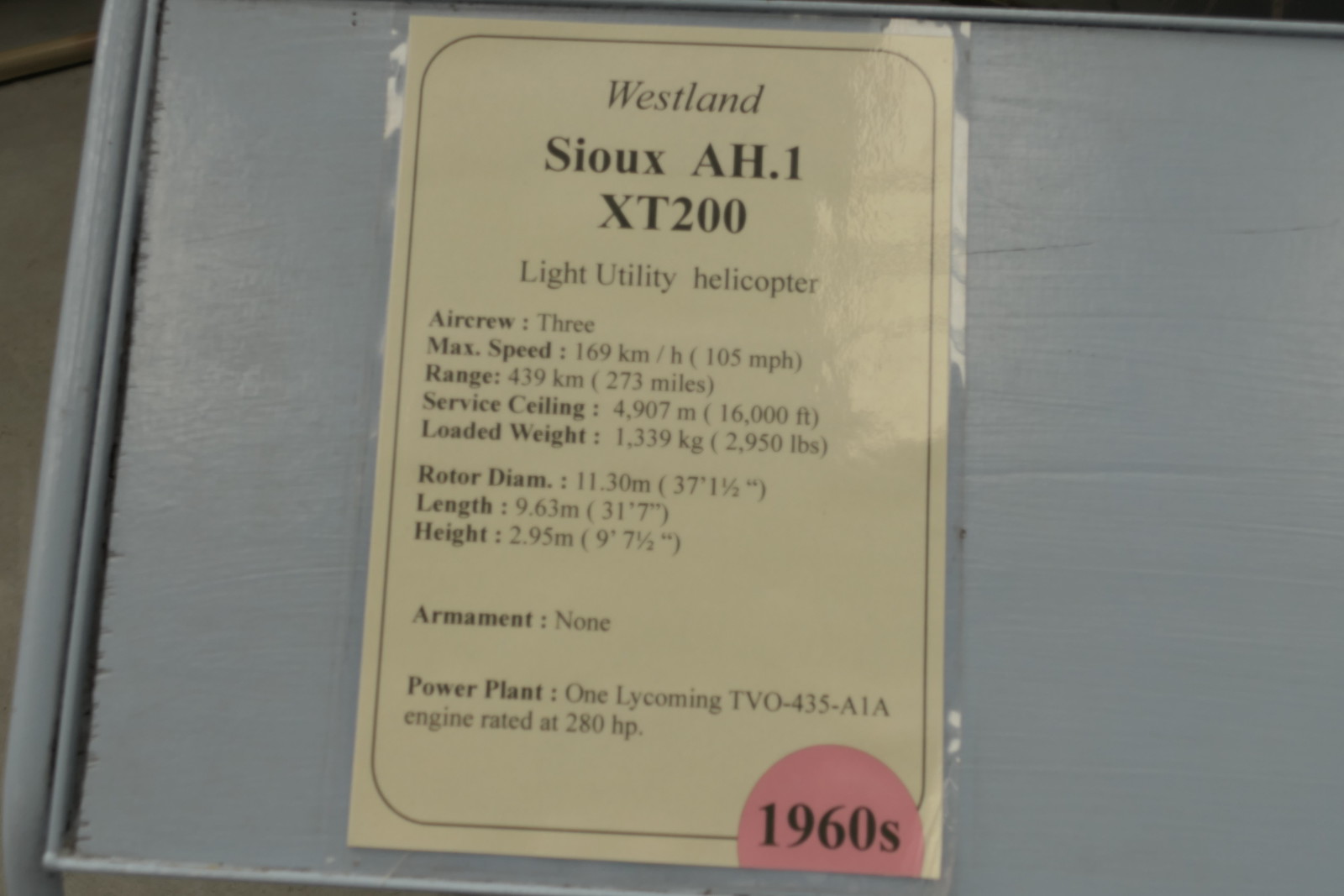The image displays a detailed sign affixed to a gray, wooden structure, possibly part of a display or museum exhibit. The off-white, laminated document features a large pink semicircle at the bottom labeled "1960s." At the top, in italicized black script, is the title "Westland Sioux AH.1 XT-200" followed by the subtitle "Light Utility Helicopter." The sign meticulously lists the helicopter's specifications: aircrew of 3, max speed of 169 KM/H (105 MPH), range of 439 KM (273 miles), service ceiling of 4,907 meters (16,000 feet), loaded weight of 1,339 KG (2,950 lbs), rotor diameter of 11.30 meters (37 feet 1.5 inches), length of 9.63 meters (31 feet 7 inches), and height of 2.95 meters (9 feet 7.5 inches). Additionally, it notes there is no armament and mentions the power plant as a Lycoming TVO-435 A1A engine rated at 280 HP. The layout features bold and italicized categories, with all specifications provided beneath each heading.